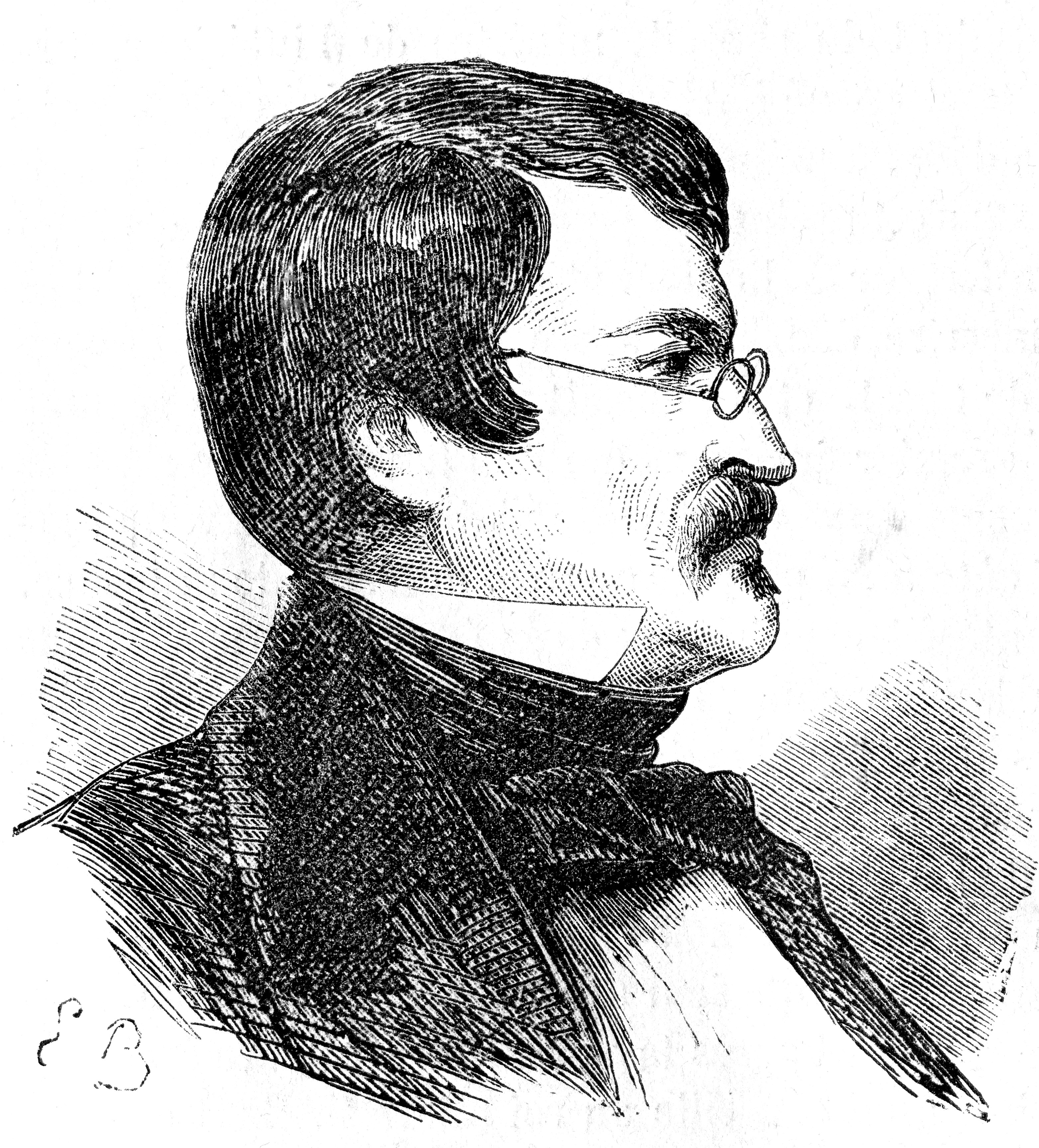This image is a highly detailed, black and white pen or pencil line drawing, possibly intended for print reproduction. It depicts a 19th-century-styled portrait of a white man in profile, facing to our right. The man has short, combed hair with distinct sideburns, and is adorned with small round spectacles perched on the bridge of his nose. His facial expression is serious and he sports a mustache. He is dressed in a professional, dark-colored jacket over a white shirt, with an upward-protruding white collar partially covered by a black collar and complemented by a black bow tie. The meticulous lines and shading exhibit a high level of detail, capturing highlights and depth. In the lower left-hand corner of the image, the letters "EB" are visible in the white space.